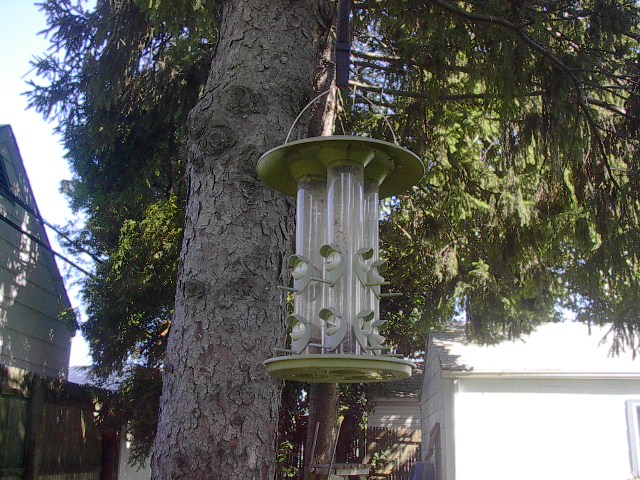In this photograph, a large bird feeder is prominently featured, hanging from the branch of a very tall, aged tree. The trunk of the tree is characterized by light brown wood with dark brown spots and rough, cracked bark, reflecting its years of growth. The bird feeder itself is green with three clear plastic tubes that contain only small amounts of bird food. Each tube has two perches and corresponding feeding holes for birds, all in green. The bird feeder is suspended amid the vibrant green leaves of the tree, through which the sunlight filters, casting varying shades of green across the scene.

In the background, to the left of the image, a tall tan house stands behind a brown fence that outlines the property. Further to the right, a brightly illuminated white building, possibly a shed or garage, contrasts against the leafy surroundings. The sun's rays peek through the foliage, highlighting the serene, backyard setting captured in the photograph.